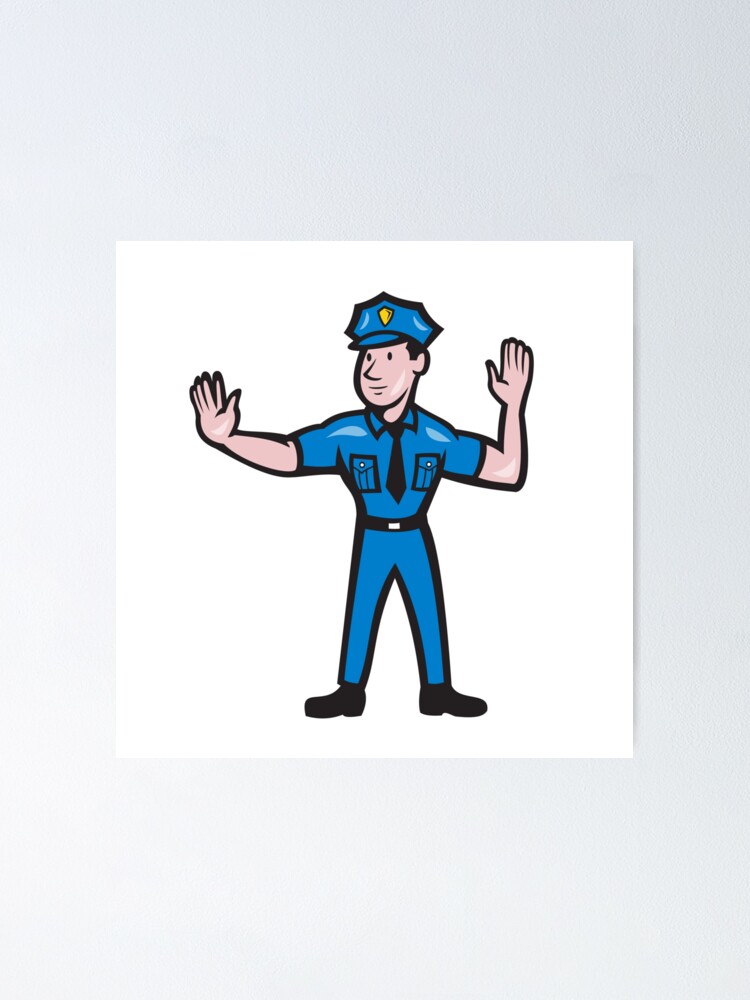This image is a cartoon-style illustration of a white police officer engaged in traffic control. The officer is depicted in a bright blue uniform, complete with a tie, black boots, and a pointed blue hat adorned with a yellow badge. He is standing with his legs slightly apart, both arms raised in a classic traffic-stopping gesture: the left hand bent at a 90-degree angle with the palm open and fingers spread, and the right hand outstretched in a similar stop-sign motion. His face shows a neutral expression, though he's slightly smiling. The drawing is set on a clean, white piece of paper, framed by a grayish-white border, giving it a "frame within a frame" appearance. The simplicity of the drawing, devoid of any detailed police equipment, reinforces its artistic, straightforward nature, capturing the essence of a traffic cop in action.